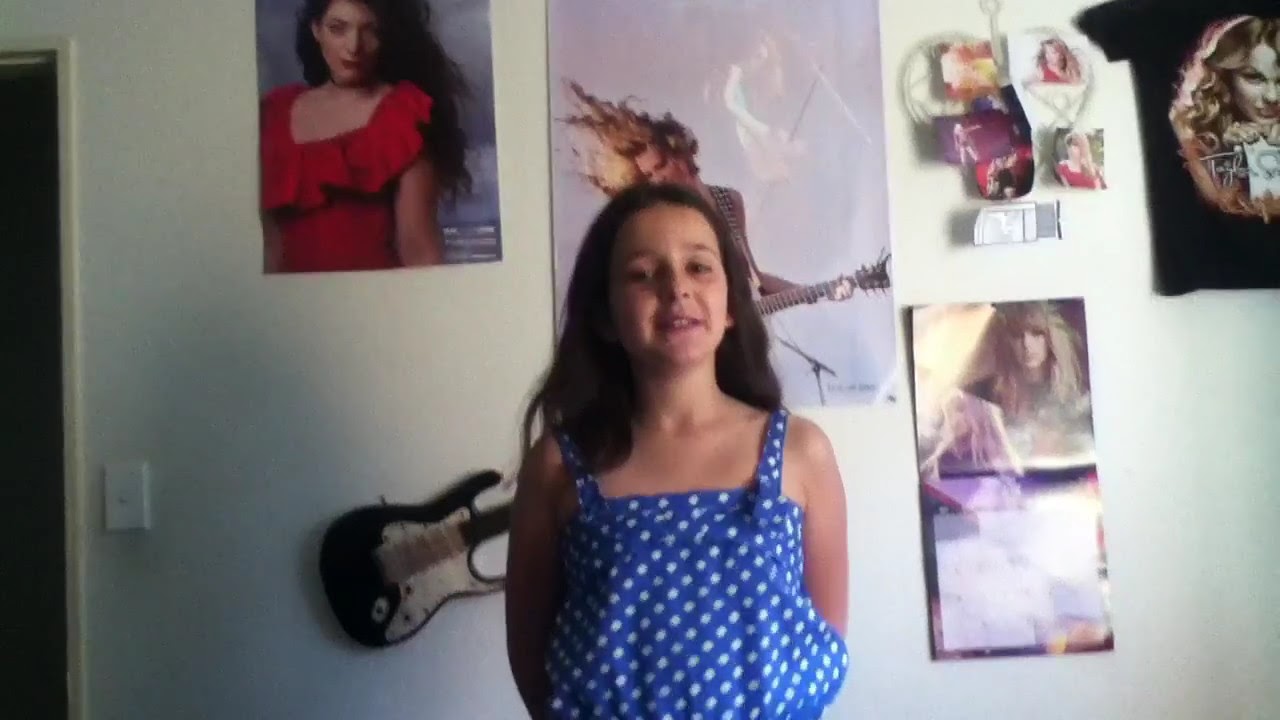In the photograph, a young girl, around 12 or 13 years old, is the main focus, standing confidently in front of what appears to be her bedroom wall. She is dressed in blue overalls with white polka dots, showcasing her unique style. Her shoulder-length dark brown hair and dark brown eyes are noticeable, and she has a neutral expression with her mouth slightly open. Behind her, the white wall is adorned with various Taylor Swift-themed decorations, indicating her admiration for the artist. 

Prominently displayed is a Taylor Swift poster, capturing the singer mid-performance with her hair dramatically flailing while playing the guitar. Below this is a Taylor Swift calendar, further emphasizing her devotion. To the right, a black Taylor Swift t-shirt is pinned to the wall, featuring the artist's photograph. Additionally, a heart-shaped collage comprises smaller pictures of Taylor Swift, creatively arranged. Just to the girl's right, a black electric guitar with a white pick guard adds a musical touch to the setting. The scene also includes a doorway to the left and a general mix of colors like blue, white, tan, beige, brown, black, gray, purple, red, and yellow, giving the impression of a cozy and personalized space.